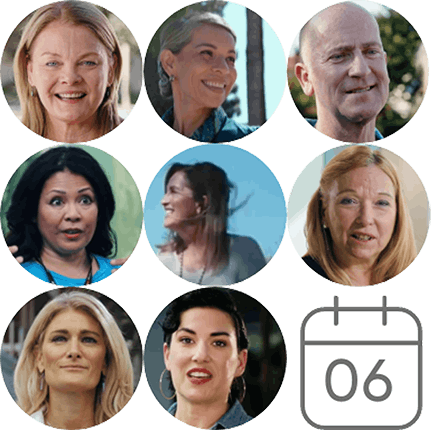The image features a white background with a 3x3 grid of circular headshots, depicting eight people—seven women and one man. The lone male, who is bald and grinning slightly, is positioned at the top right. The women appear to be middle-aged, ranging from their 40s to 50s, and exhibit a variety of expressions; most are smiling, while others look surprised or are glancing away from the camera, giving a professional yet diverse feel to the group. At the bottom right corner of the image, there's a grey, rounded square graphic resembling a calendar showing the number "06," suggesting a date. This composition could represent participants for a meeting scheduled on the 6th of the month, possibly displayed within a smartphone app for colleague identification and meeting organization.